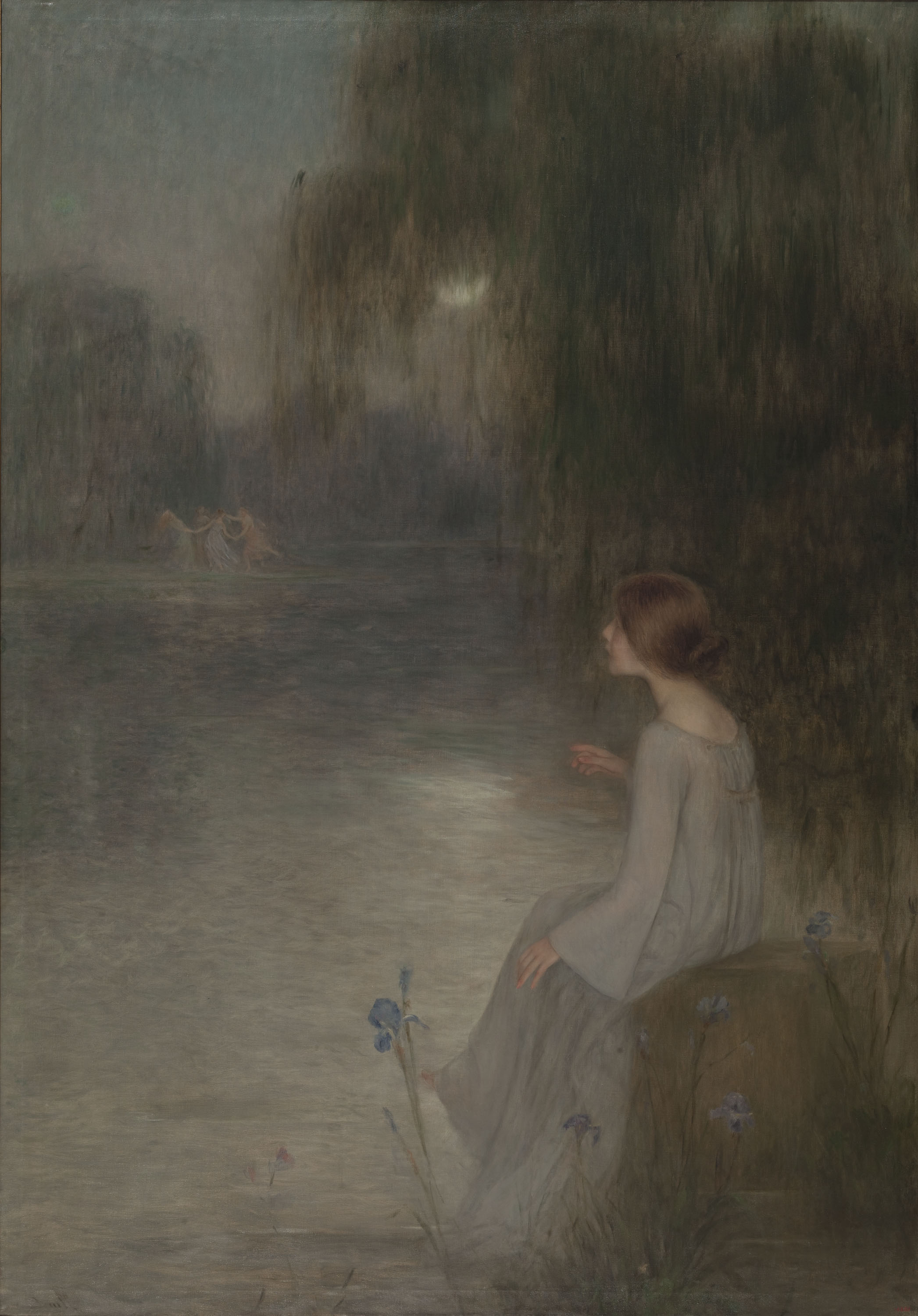This oil painting, titled "Somni" by Joan Brull, is a Romanticism piece created in the late 1800s. The painting, in portrait orientation, depicts a somewhat blurry, muted, and misty night scene, reminiscent of a white night due to the subtle light in the sky and the visible crescent moon. In the bottom right corner of the piece, a young woman with white skin and medium brown hair styled in a bun sits on a rock or a brown chest near a grayish pond. Dressed in a long, light gray or white gown, she gazes across the moonlit water with her right hand raised, revealing only her side profile to the viewer.

Surrounding the serene pond are trees, including a prominent willow tree to the right behind the woman, and blue irises in the foreground near her. In the distance across the water, a group of women in long colorful gowns dance in a circle, holding hands in the moonlight. The calm, reflective water and the embracing foggy atmosphere add to the painting's ethereal and dreamlike quality.